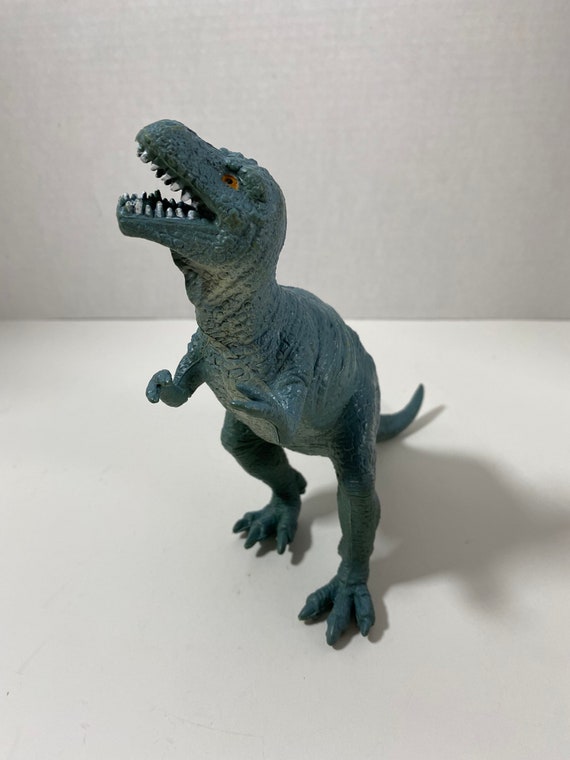This is a detailed photograph of a toy dinosaur, specifically a T-Rex, set against a white background. The T-Rex has a teal-tinged, dark bluish-gray body with short, claw-like forearms characteristic of a predator. Notable features include its sharp white teeth, which are visible as the dinosaur’s jaws are slightly agape. It has a striking orange eye with a black pupil, giving it a menacing appearance. The head is turned to one side, allowing only one eye to be visible, while the body faces more towards the camera. The dinosaur's underbelly and neck transition to a pale yellow shade, adding to its realistic detailing. The figure is posed against a white background, where the separation between the wall and the floor is visible. There is also a shadow cast to the bottom right, suggesting a light source from the top left. The feet of the toy are thicker and darker in color with less texture detail, adding depth to the overall impression of the toy.